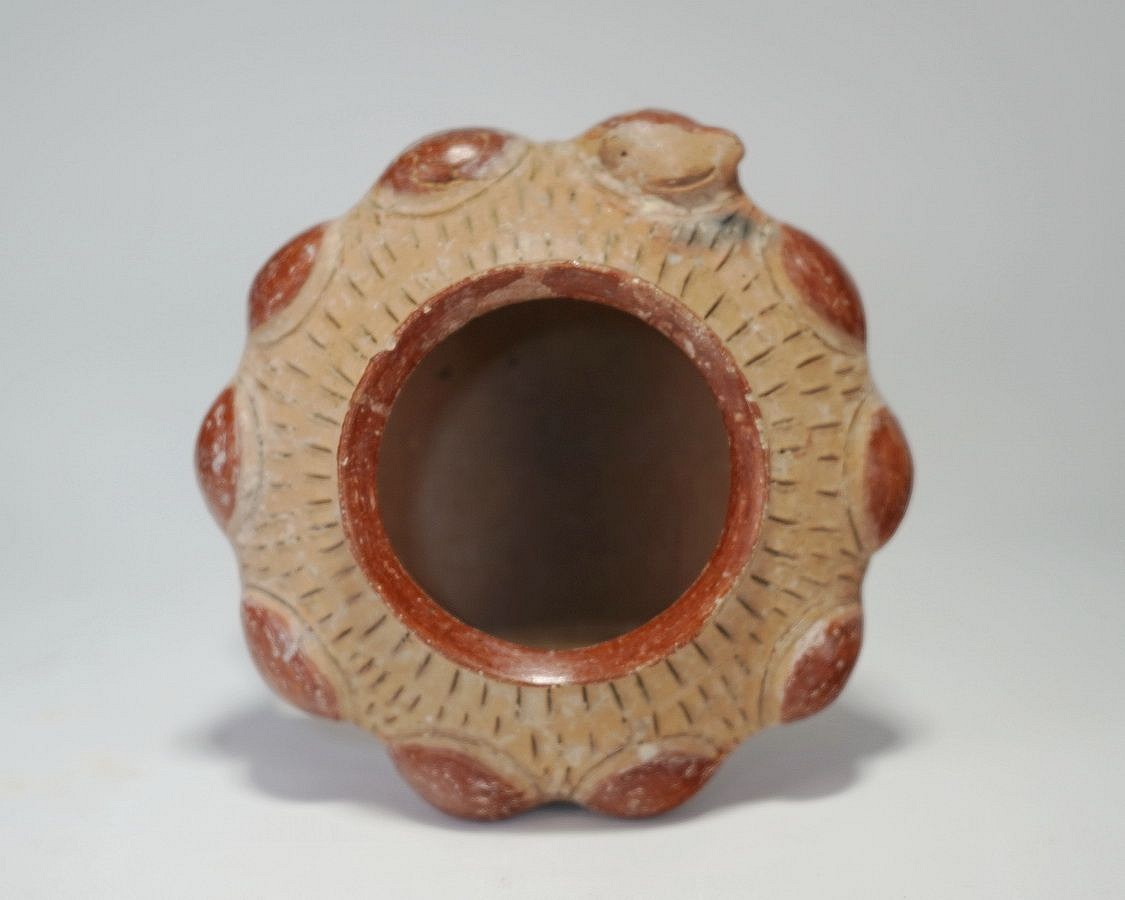This photograph showcases a handmade clay artifact, prominently centered against a stark white gallery-like backdrop. The object is round with an irregular edge, featuring numerous raised, scalloped bumps uniformly spaced around its circumference. These bumps are painted a distinct red color that contrasts with the primary beige and dark orangish-brown hues of the piece, which also include subtle black flecking. At its hollow center, the artifact reveals a deep red circle with a glossy, reflective black tint, suggesting a glass-like finish. The intricate craftsmanship and textural details underscore its unique and artistic nature.